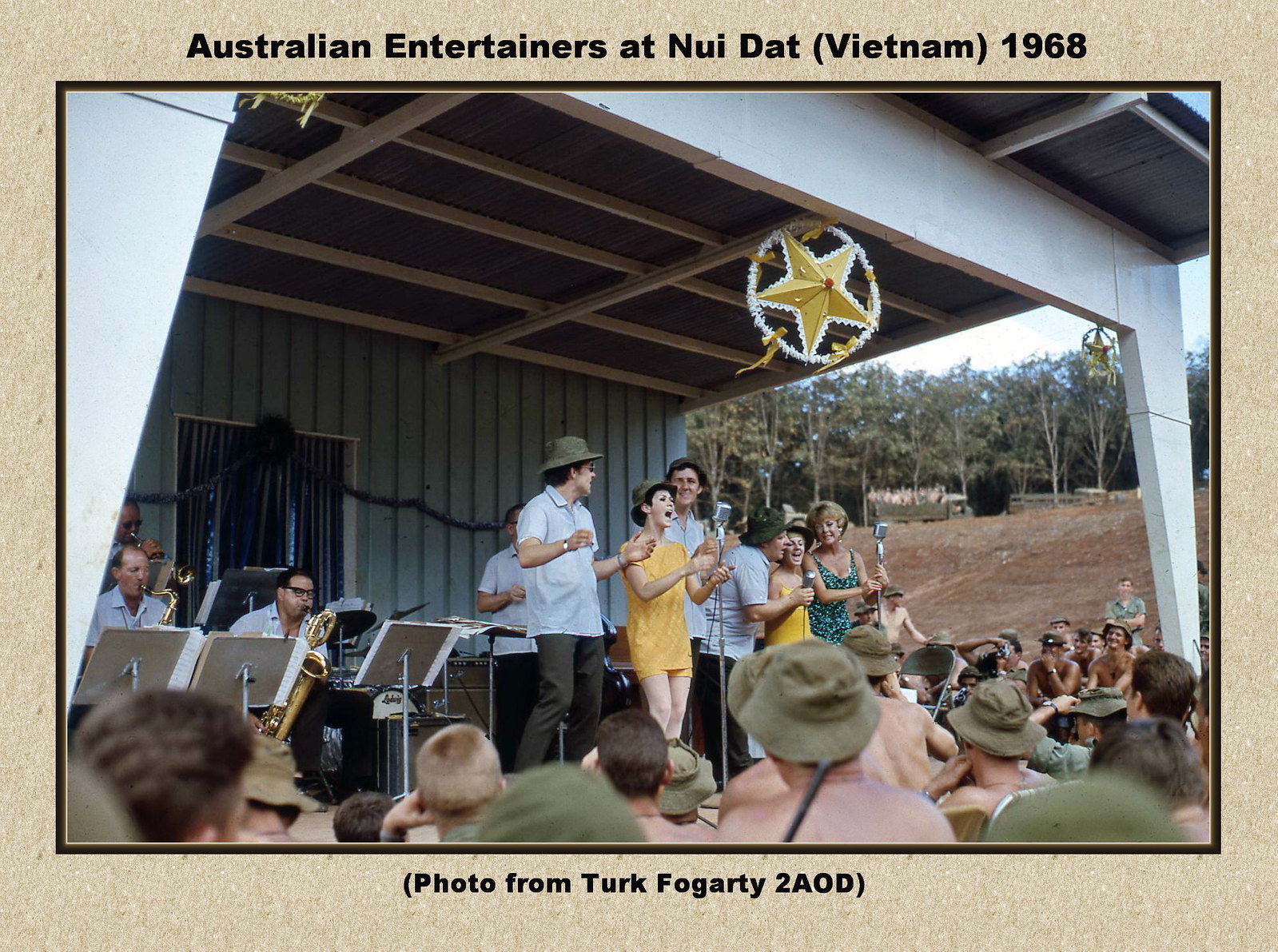The image depicts a lively performance by Australian entertainers at Nui Dat, Vietnam, in 1968, showcased within a brown-bordered photograph captioned "Australian Entertainers at Nui Dat, Vietnam, 1968," with credits to "Photo from Turk Fogarty, 2-A-O-D" at the bottom. Dominating the wooden stage, adorned with vertical slats and a prominent gold star surrounded by a white wreath on its top front, the scene captures a central female vocalist dressed in a matching yellow shirt and shorts ensemble, singing into a vintage silver microphone. Flanking her are several other performers, including two additional female singers to the right and men in green bucket hats and blue collared shirts. The background reveals an orchestra with musicians handling horns, including trumpets and saxophones, indicating a well-rounded musical setup. In the foreground, the audience consists mostly of shirtless military personnel wearing green hats, some seated on a hill to the stage's right, with trees and a sprawling field visible in the distance.